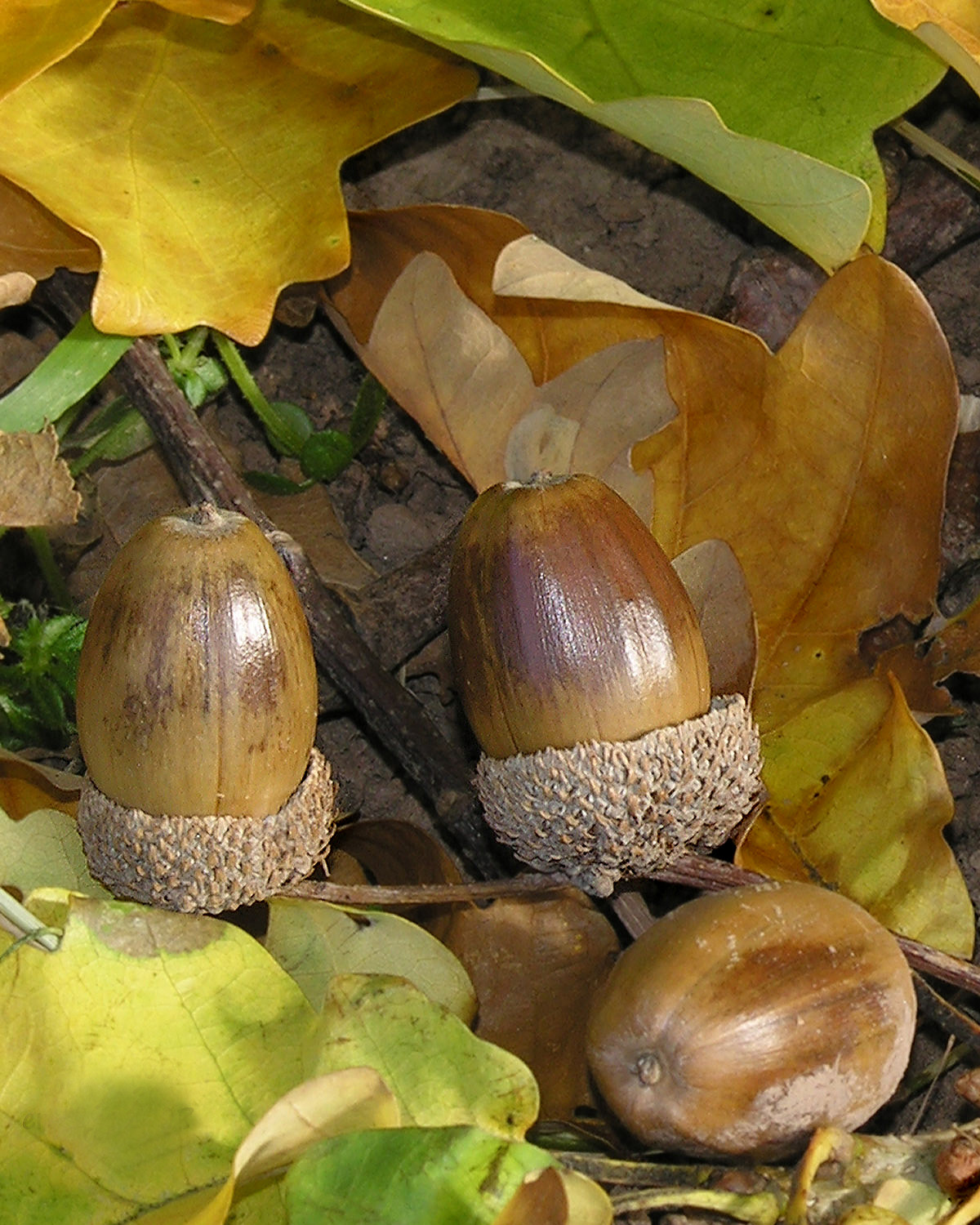This high-quality, close-up color photograph showcases a detailed arrangement of three acorns that have fallen onto the ground, two of which retain their caps. The acorns are nestled amidst a layer of light brown, curled, and crunchy leaves, with additional yellow, green, and orange leaves scattered around, adding a vibrant contrast. Some of the leaves are casting subtle shadows on the soil beneath, which is interspersed with both broken and intact brown twigs and branches, creating a rich tapestry of natural elements. The overall clarity and detail suggest the use of a professional-grade camera, capturing the intricate textures and hues of this autumnal scene.